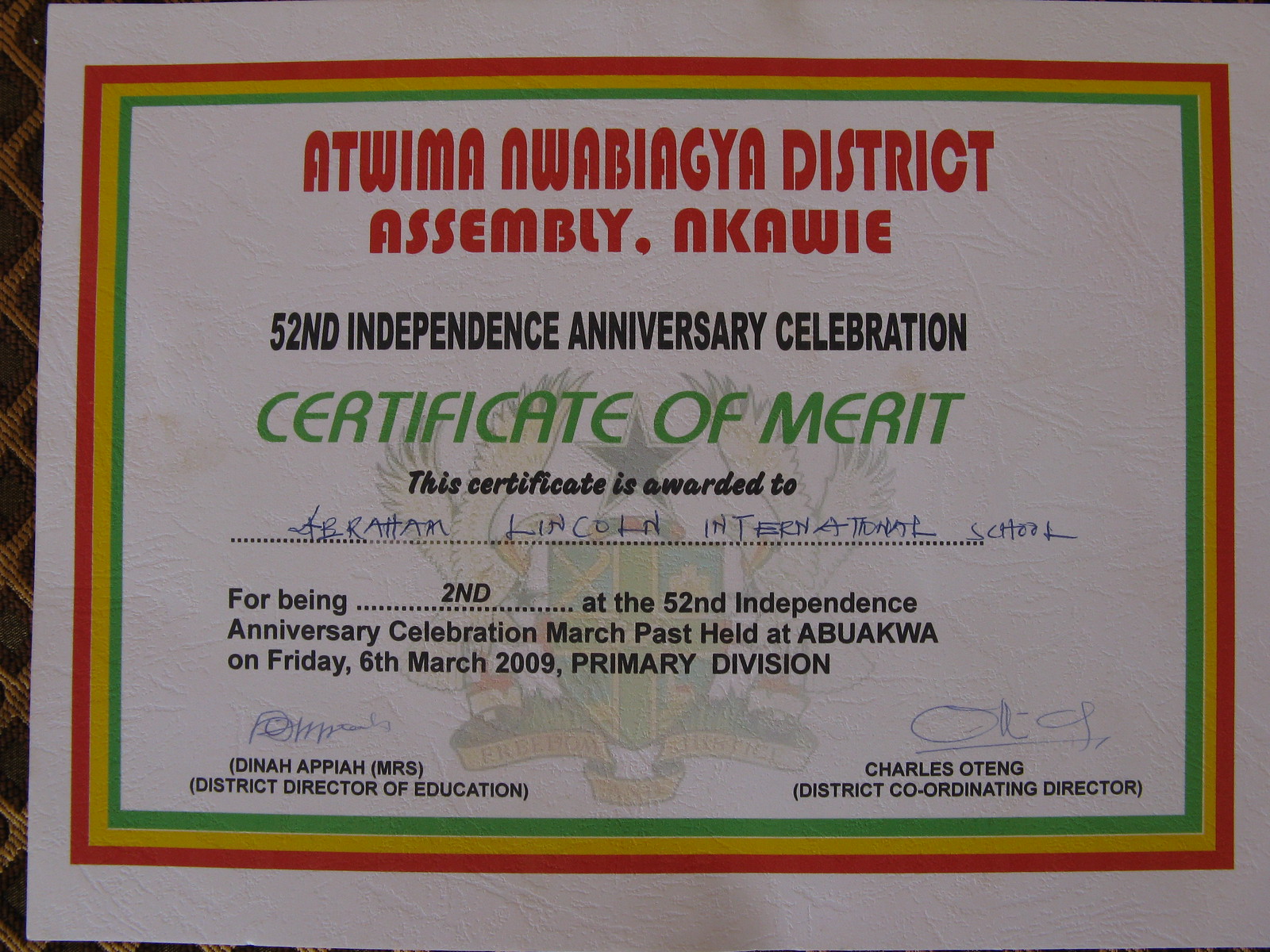This photograph showcases a highly detailed Certificate of Merit awarded by the Atwayma Nwabekia District Assembly to Abraham Lincoln International School. Commemorating the 52nd Independence Anniversary Celebration, the certificate acknowledges the school for achieving second place in the March Past event held at Abu Aqua on Friday, 6 March 2009. The certificate's professional design features a white background framed by bold red, yellow, and green borders. Centered meticulously, the text begins with "Certificate of Merit" in prominent red font, followed by black, green, and more black text detailing the event and award. Handwritten in blue ink are the awarded details and signatures. The layout includes a faint, translucent plaque-like logo that adds a touch of sophistication without overwhelming the visual simplicity. The overall aesthetic is marked by its minimal color scheme and elegant typography, making it appear very important and prestigious.